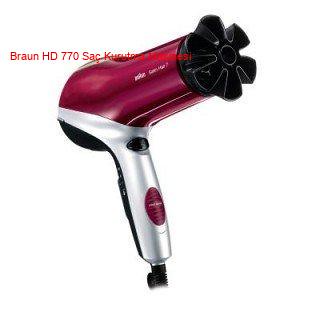The image displays a realistic photograph of a hairdryer, set against a pure white background that appears either digitally edited or taken specifically this way for a catalog. The hairdryer is prominently marked with red text that reads "Braun HD 770 SAC" and another unlegible term. The device features a sleek design with a variety of colors: a white and silverish handle with a red button and a black button, a black back, and a black extension cord at the bottom. The barrel of the hairdryer is a purplish red color, ending in a unique black nozzle shaped like a six-sided star or an exaggerated daisy with a hollowed-out center. Additionally, there is white lettering on the red body of the hairdryer. This detailed visual representation emphasizes its appeal for potential buyers and highlights its placement in commercial catalog imagery.